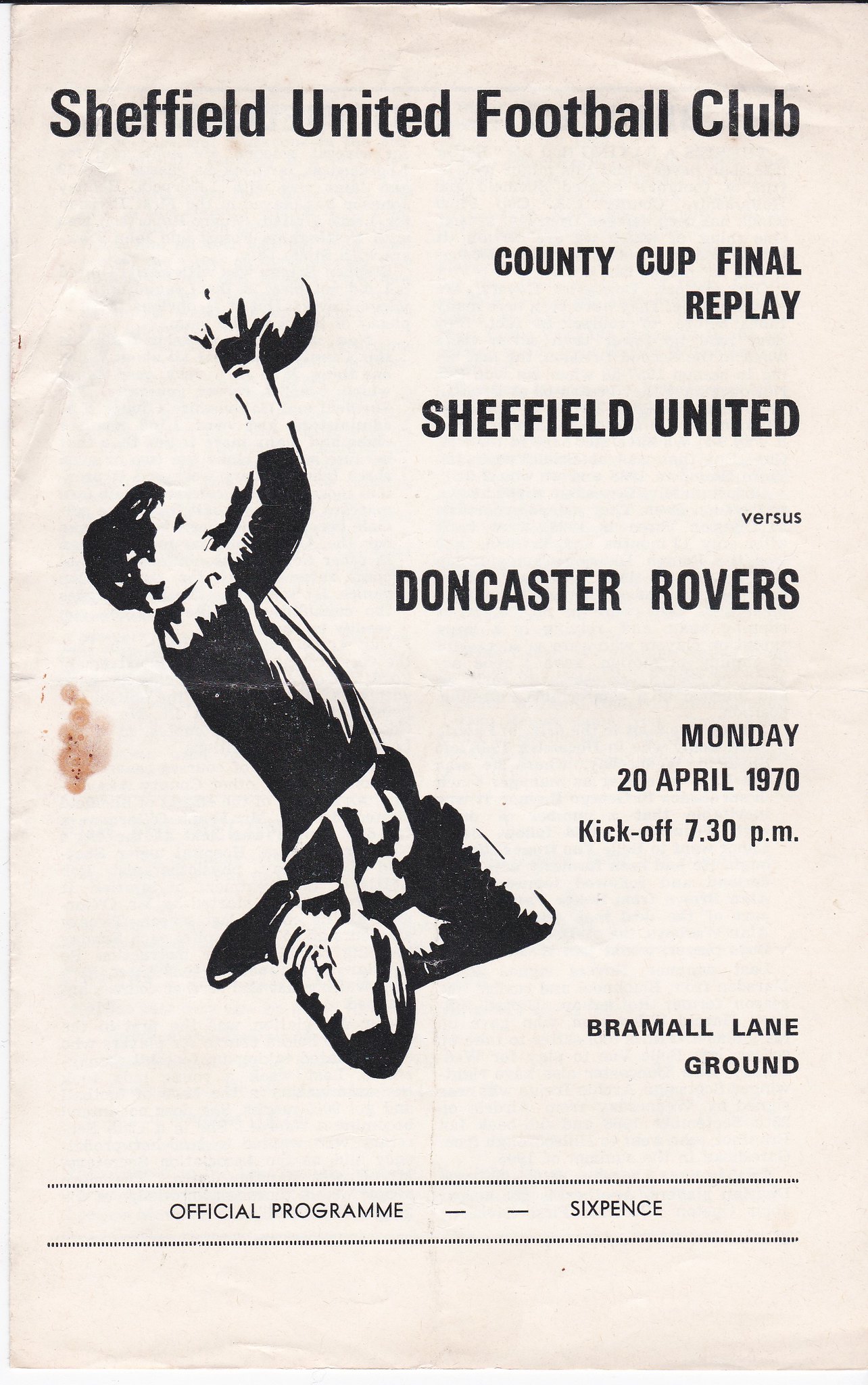This single-page, portrait-oriented image is the official program for a historical soccer match, prominently featuring a vintage, black-and-white design. At the top in bold black text, it announces, "Sheffield United Football Club." Below this header, aligned on the right, it details the "County Cup Final Replay" between "Sheffield United versus Doncaster Rovers," scheduled for "Monday, 20 April 1970," with a kickoff time of "7:30 p.m." at "Bramall Lane ground." The bottom of the page features a horizontal band that reads, "Official Program," with the cost of "Sixpence." On the left side, capturing the viewer's attention, is a black-and-white illustration of a goalkeeper jumping to catch a ball, adding a dynamic visual element. The color scheme includes shades of tan, black, gray, and a faint hint of brown, contributing to its nostalgic, vintage print style. The positioning of text and imagery suggests it's a classic memorabilia piece from a British football club's past event, encapsulating the era's program design.